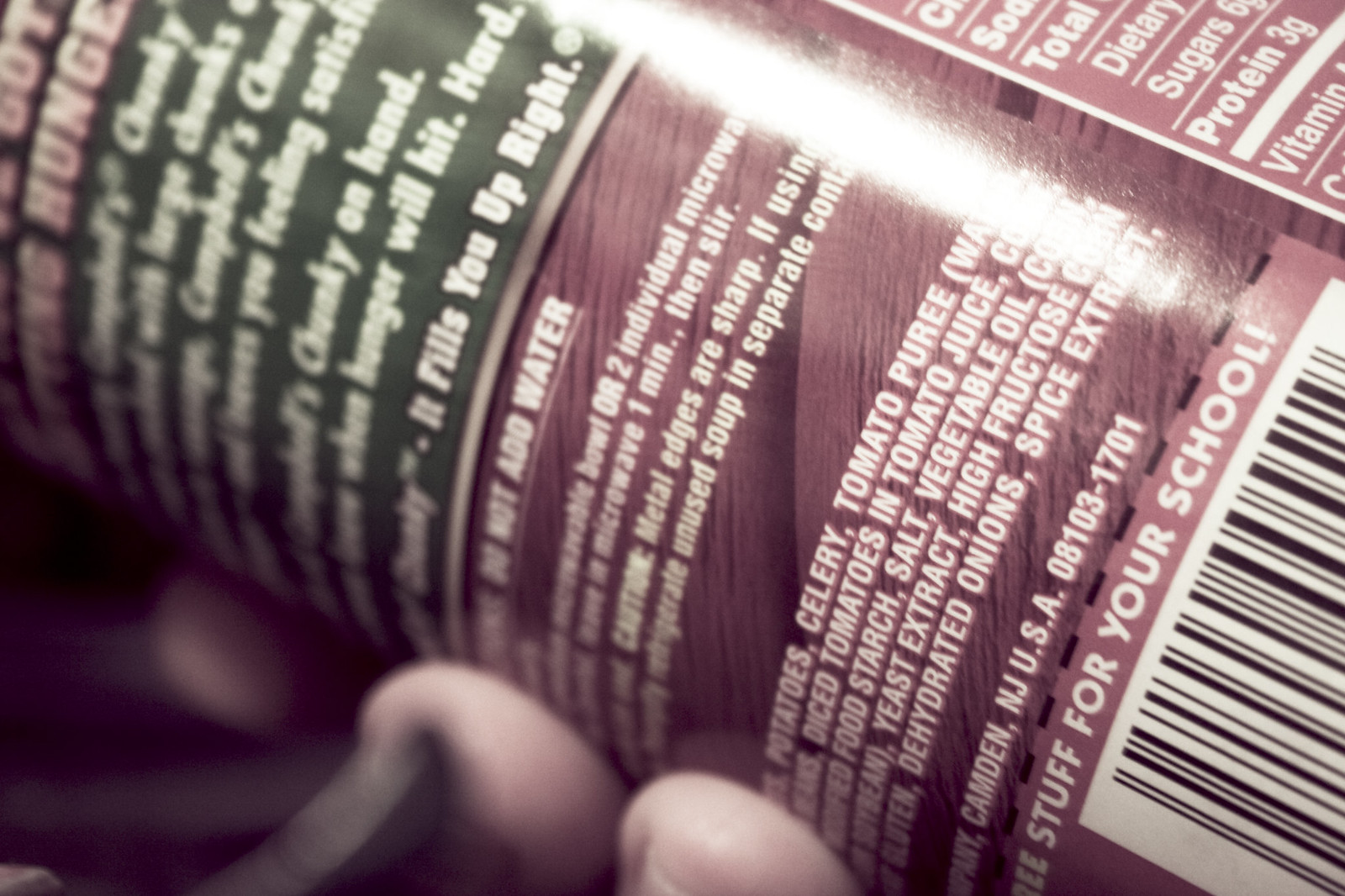A close-up image features a can of Campbell's soup, held in someone's hand. The photo focuses on the back label of the can, making it impossible to identify the specific type of soup from the front. The label prominently mentions phrases such as "hunger" and "chunky, large chunks," suggesting its hearty, filling nature. Additional text highlights that the soup is designed to leave you feeling satisfied, emphasizing the "chunky" aspect. The label advises not to add water and cautions against sharp metal edges. It also provides storage instructions, recommending refrigeration of unused soup in a separate container. The ingredients listed include potatoes, celery, tomato puree, tomatoes and juice, vegetable oil, salt, starch, yeast extract, high fructose corn syrup, spices, hydrated onions, and more. The bottom portion of the label displays a white and black line barcode.